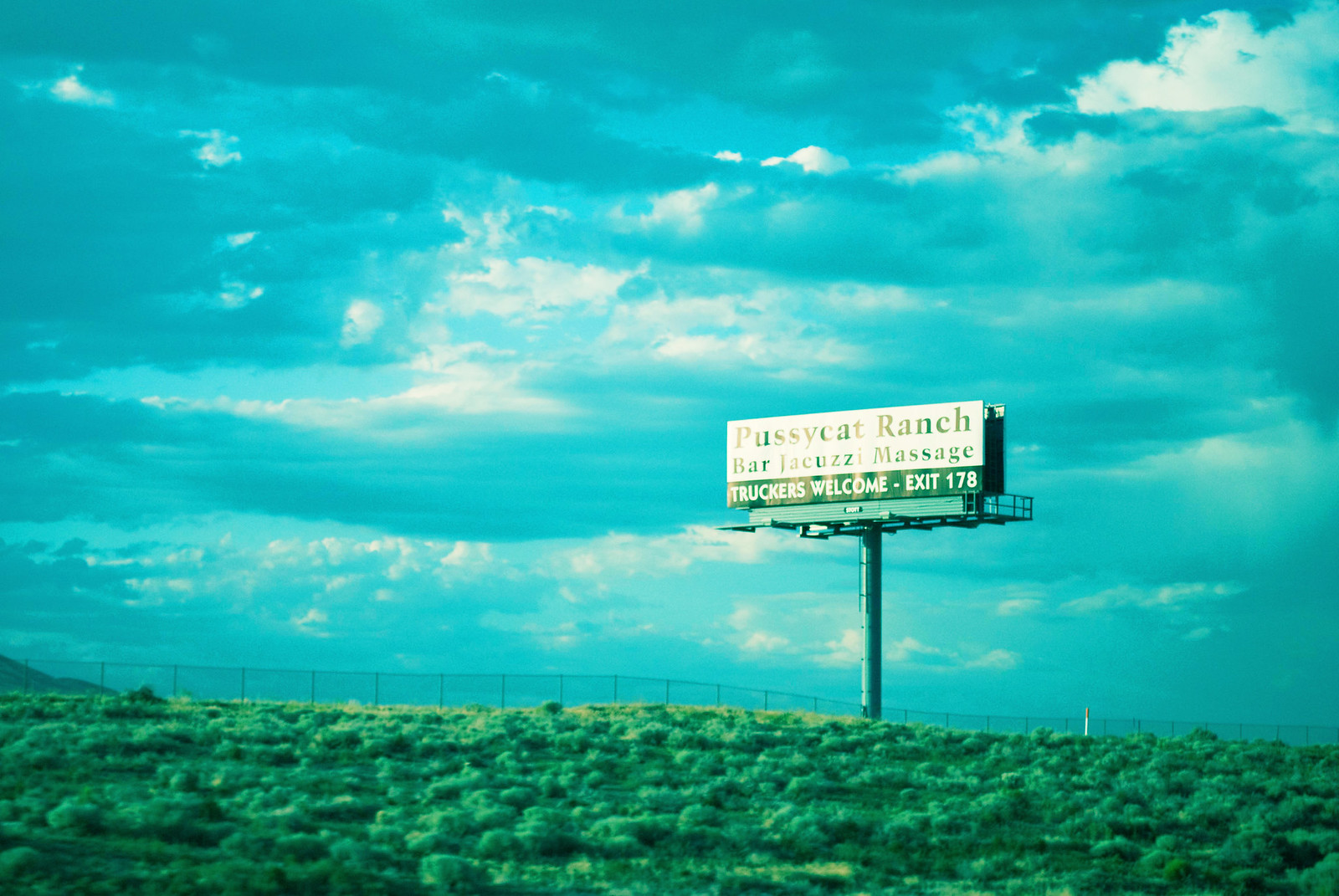This vibrant color photograph captures an expansive desert landscape, characterized by its arid terrain speckled with various desert shrubs and tumbleweeds. In the mid-ground, a chain-link fence stretches horizontally across the image, creating a stark boundary between the rugged foreground and the objects beyond. Dominating the scene beyond the fence is a large, weathered billboard, positioned to attract the attention of travelers. The sign advertises "Pussycat Ranch Bar Jacuzzi Massage," welcoming truckers and directing them to exit 178. The distant road implied by the billboard remains out of sight. Overhead, the sky is a dramatic tapestry of gray and white clouds, adding a sense of depth and moodiness to the composition.